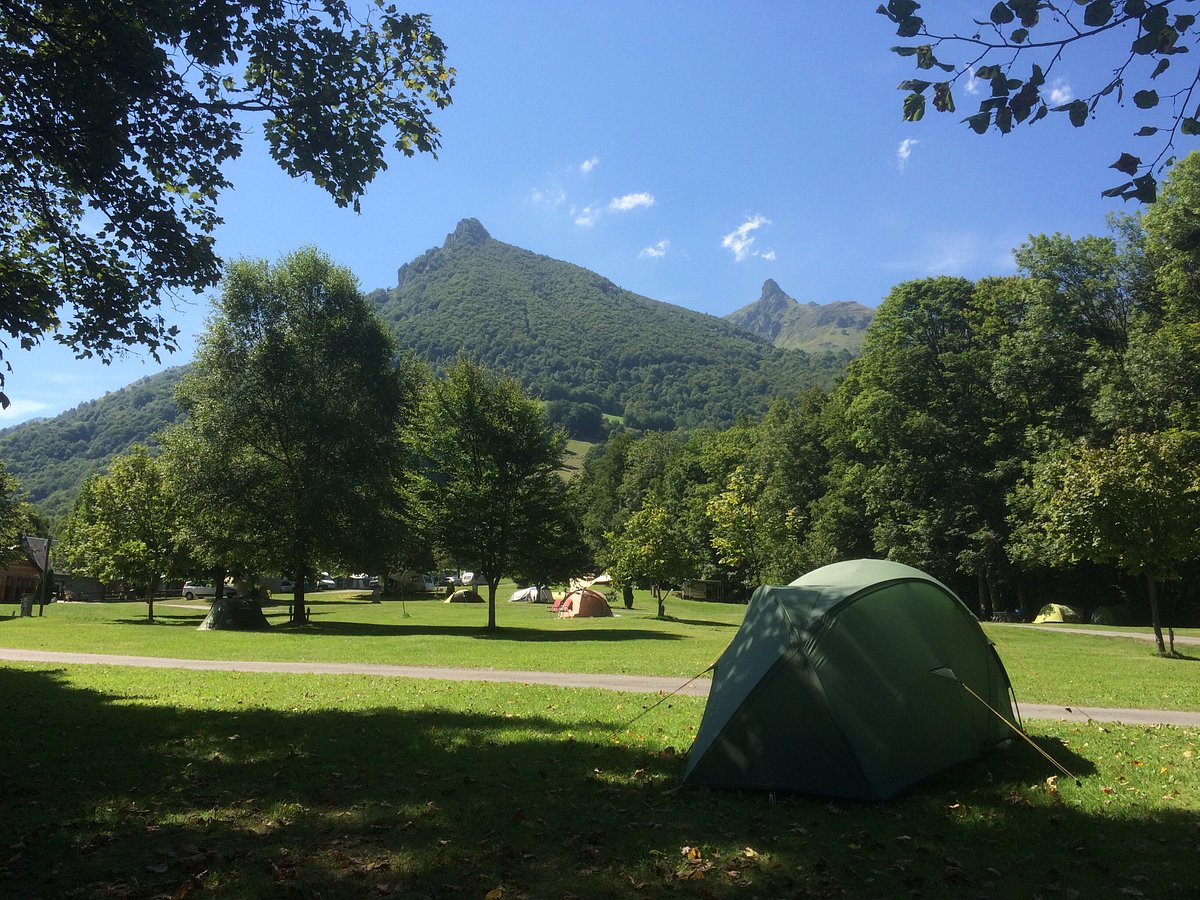The image depicts a vibrant campsite set on a meticulously maintained lawn under a sunny, clear sky with a few scattered clouds. Shadows cast by the surrounding trees indicate bright sunshine. Multiple tents dot the area, including a prominent green dome tent in the shady foreground and others like a yellow tent to the right, and an orange and white tent further in the distance. A paved footpath bisects the green expanse, adding structure to the scene. This natural setting is completed by a lush, forested mountainside in the background. The site is well-organized, with no people visible, and hints of civilization, such as a small white car and other vehicles, suggest proximity to a car park. A building can also be seen in the background, integrating man-made elements with the natural tranquility of the campsite.